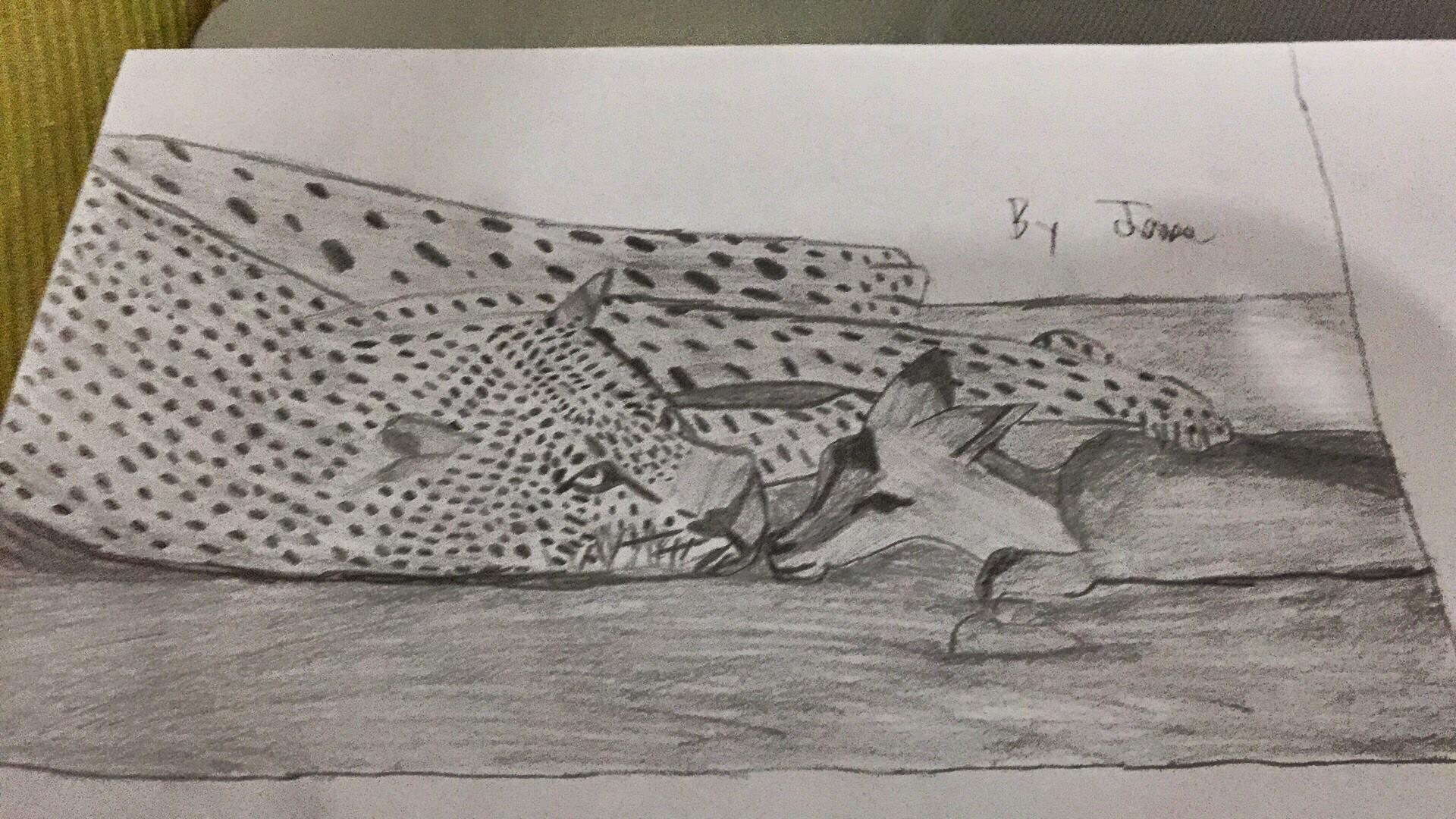A black-and-white drawing lies on a table, neatly captured in a photograph. The artwork depicts a leopard and a fawn in a striking and stylized manner. The leopard is shown lounging with its legs outstretched, its head resting on the floor, and its nose nearly touching that of the fawn. The fawn, contrastingly, has a body that is more abstract and stylized, though the attempt to approach realism is evident in both figures. The surreal nature of the scene is poignant, given that such a peaceful interaction between predator and prey is highly unlikely in reality. The intricate details of the drawing, combined with its artistic flair, evoke a sense of delicate harmony between the two animals.